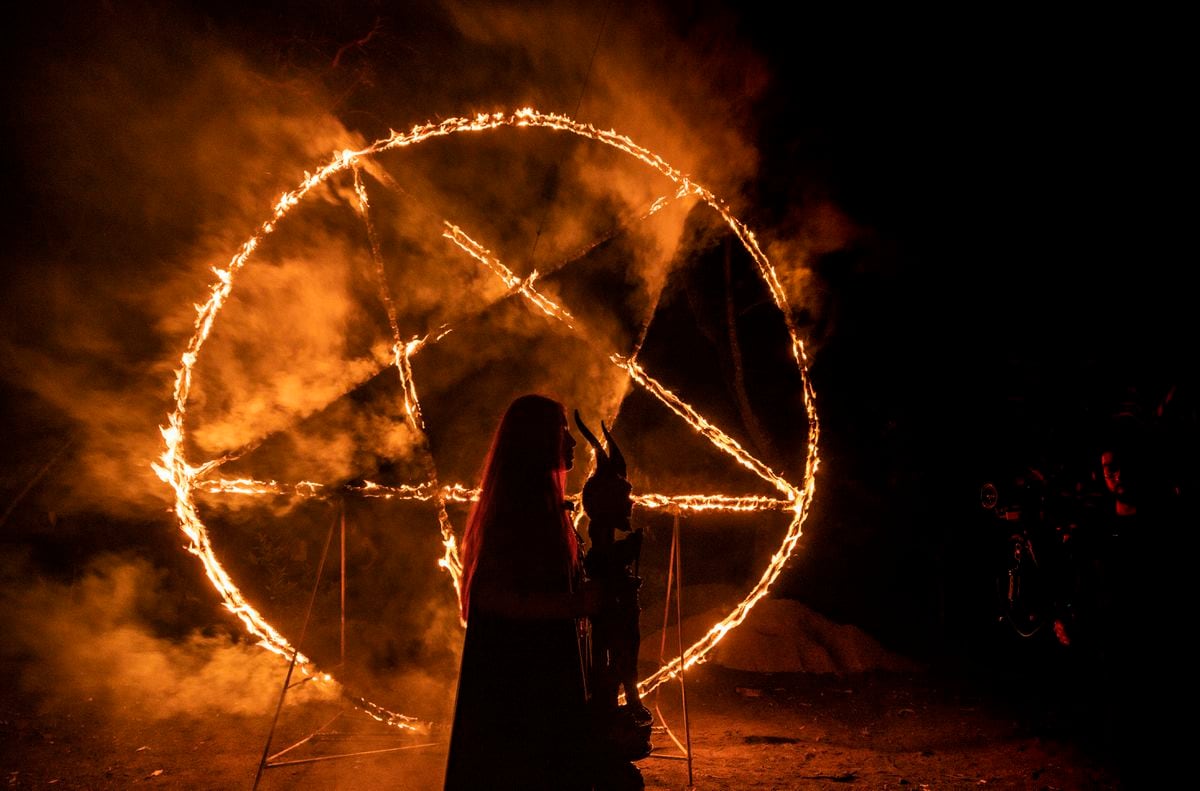The horizontal rectangular image vividly depicts a dramatic scene involving a fiery symbolic ritual. Dominating the center is an intricate golden circle with intersecting lines forming a pentagram, which appears engulfed in flames and emanating dense smoke. The burning symbol casts an intense orange hue across its surroundings, contrasting sharply with the dark background that envelops the rest of the image. 

At the forefront stands a figure, likely a woman inferred from her long, seemingly red hair due to the fiery reflection. She is clad in a long black robe and appears to be holding a hand to her head. The woman cradles an object that resembles a stuffed animal, possibly a rabbit, evoking imagery akin to the one from "Donnie Darko." Another significant detail is that the object she holds also has two prominent pointed horns, suggesting a statue rather than a plush toy.

The ground beneath them looks rough, possibly gravel or sand, adding a raw texture to the scene. To the right, there is another figure who might be holding a camera, insinuating that this intense and mysterious event is being documented. The stark contrast between the glowing, fiery central motif and the otherwise black surroundings amplifies the ritualistic and possibly demonic undertones of the image.